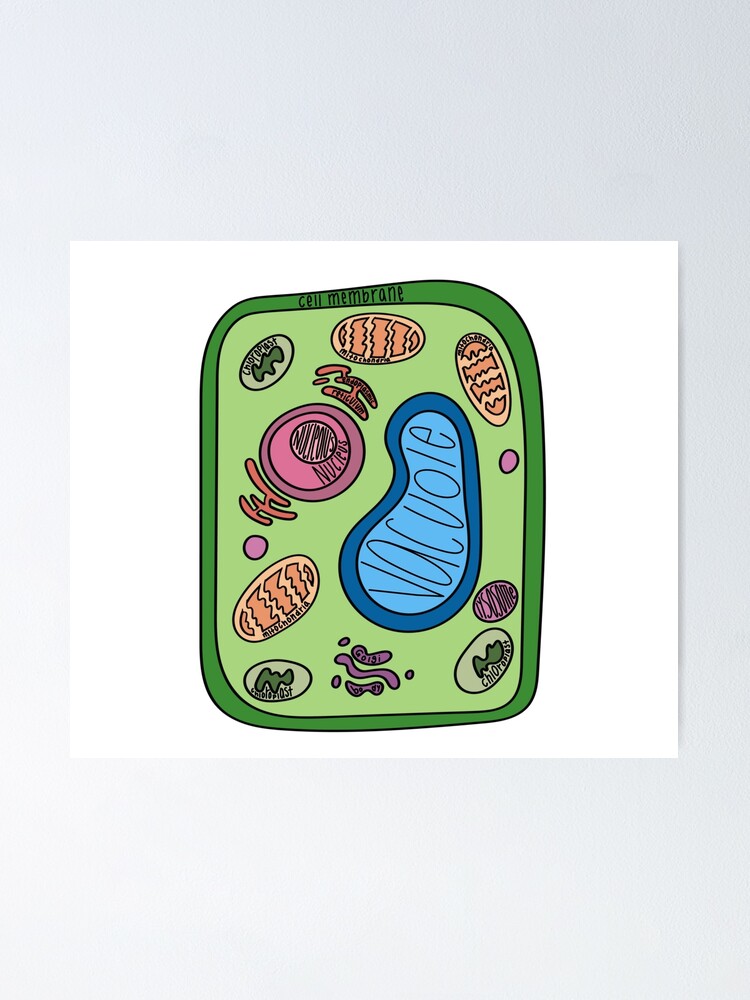The rectangular image, measuring approximately six inches high and four inches wide, is a detailed drawing of a cell against a white background, encased in a dark green border. At the top, the label “cell membrane” appears in black font. Inside the border, the cell itself features a light green background populated with various cellular structures, each distinctly marked. The central large, blue, peanut-shaped object is labeled "vacuole." Three light green ovals, each labeled "chloroplast," are dispersed within the cell. There are three egg-shaped, orange objects marked "mitochondria," characterized by internal zigzag lines. Additionally, a small pink oval labeled "isotope" and a large pink circle with the label "nucleus" are present. Finally, scattered throughout are red elongated objects marked "endoplasmic reticulum." The cell membrane surrounds these components, encapsulating the intricate inner world of this biological cell diagram.